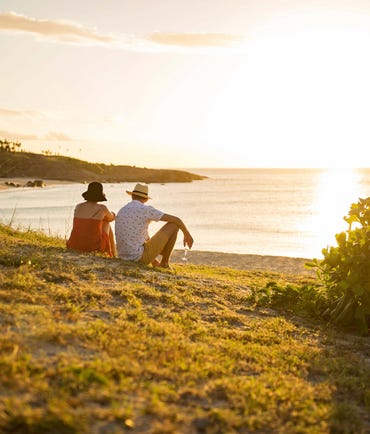In this serene and somewhat grainy picture, two adults are sitting on a beach-like area, gazing out over calm, clear water. The man, wearing a straw Panama hat, a white printed shirt, and khaki shorts, holds a wine glass in his right hand. The woman beside him, with a dark brown hat, is dressed in an orange spaghetti-strap dress. Despite some blurriness, the image captures the peaceful atmosphere of the setting, which includes green growth sprouting from the sandy ground around them. Behind them, to the left, is a patch of green land. The skies are bright with few clouds, suggesting a pleasant, enjoyable day perhaps nearing sunset. In the distance, a faint silhouette of a boat blends into the horizon, adding to the calmness of the scene.